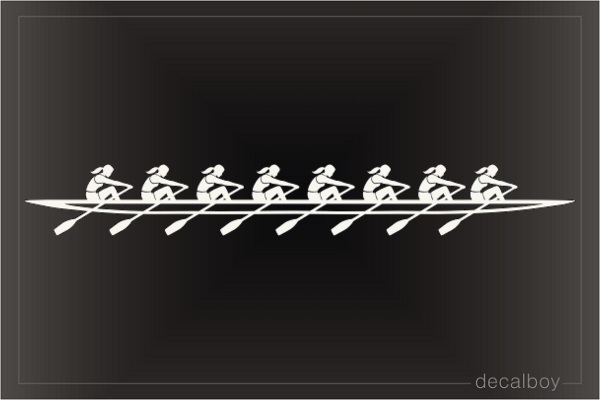The image is a black-and-white decal featuring a long canoe with eight rowers, all of whom appear to be women with ponytails. They are depicted as white silhouettes against a predominantly black background, adding a stark contrast that highlights the fine line work of the illustration. Each rower is dressed in short-sleeved shirts and shorts, outlined in black, and positioned in unison with their oars facing towards the viewer, indicating synchronized rowing towards the right. The canoe runs horizontally through the center of the image, creating a rhythmic pattern of repetitive figures. The entire design is encased in a thin white border, and at the bottom right corner, the text "decal boy" is displayed, completing the minimalist yet detailed composition.